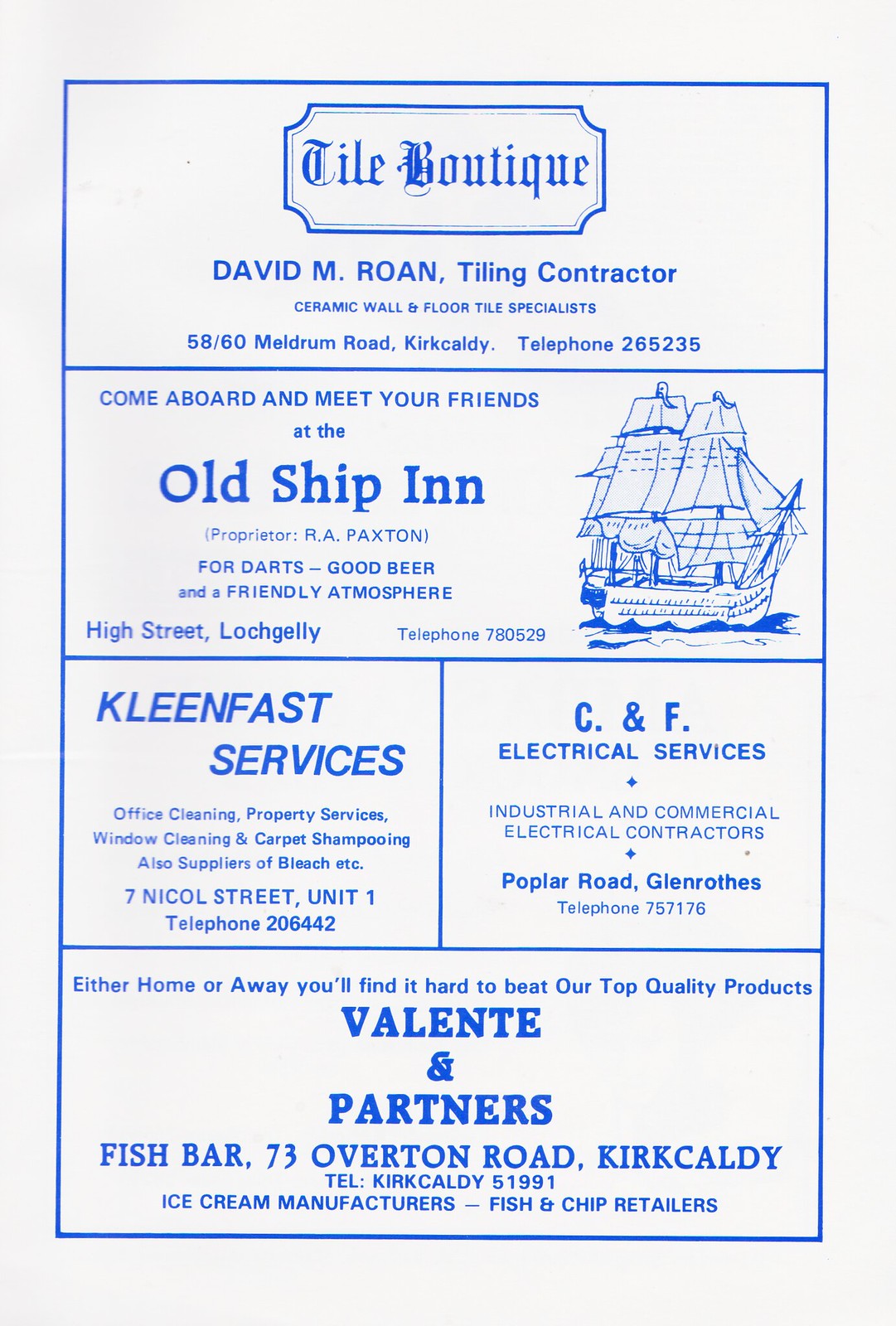This image appears to be a page from an official program, possibly from a soccer game, filled with various advertisements. At the top, there's an ad for "Tile Boutique" featuring David Amarone, a tiling contractor and ceramic wall and floor tile specialist, located at 58/60 Meldrum Road, Kirkcaldy, with contact number 265-235. Next, there's a full-width advertisement inviting readers to "Come aboard and meet your friends at the Old Ship Inn," managed by proprietor R.A. Paxton. The inn offers darts, good beer, and a friendly atmosphere on High Street, Luckgilly, phone number 780-529. Another ad features "Clean Fast Services," which offers office cleaning, property services, window cleaning, and carpet shampooing, and supplies bleach and other products, located at 7 Nicoll Street, Unit 1, with telephone number 206-442. Adjacent to this is an ad for "CNF Electrical Services," industrial and commercial electrical contractors located on Poplar Road, Glenrose, with contact number 757-176. Lastly, at the bottom of the page, a wide advertisement for Valente and Partners, a Fish Bar located at 73 Overton Road, Kirkcaldy, phone number Kirkcaldy 51991, promoting their high-quality products both locally and for takeaway, including their services as ice cream manufacturers and fish and chip retailers.